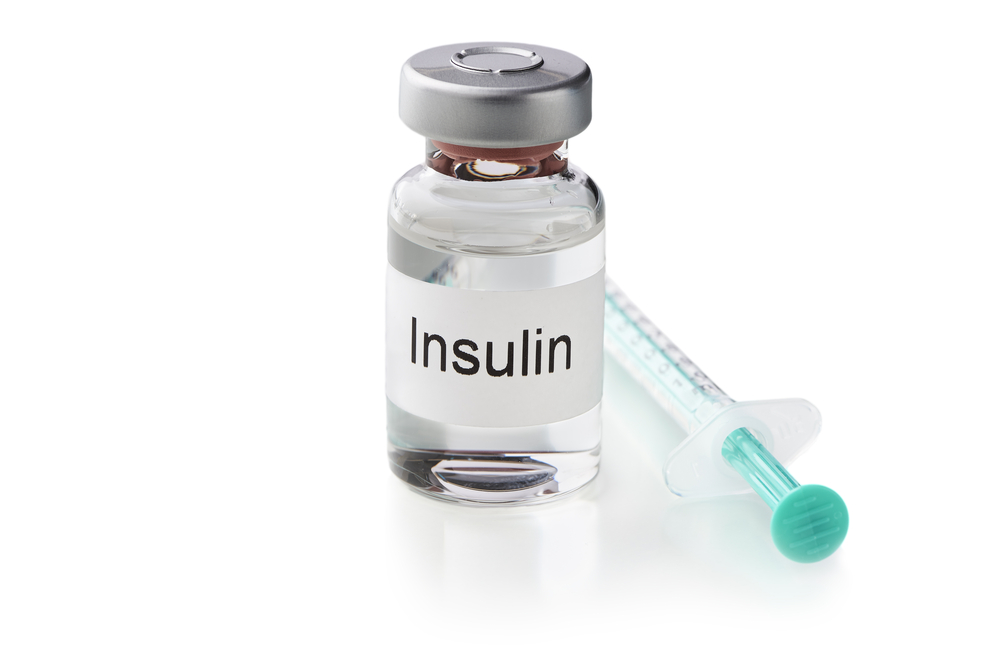This image depicts a detailed and edited photograph of an insulin bottle and an administering needle laid out on a plain white background. The insulin bottle, which is standing upright, features a grey steel cap and is filled with a clear liquid. It is wrapped with a white label that prominently displays the word "insulin" in black text. Adjacent to the bottle, the insulin needle lies horizontally, showcasing its transparent body and green plunger. The needle's handle faces towards the viewer. The photograph is minimalistic, with no additional objects or text present except for the single word "insulin" on the bottle's label.